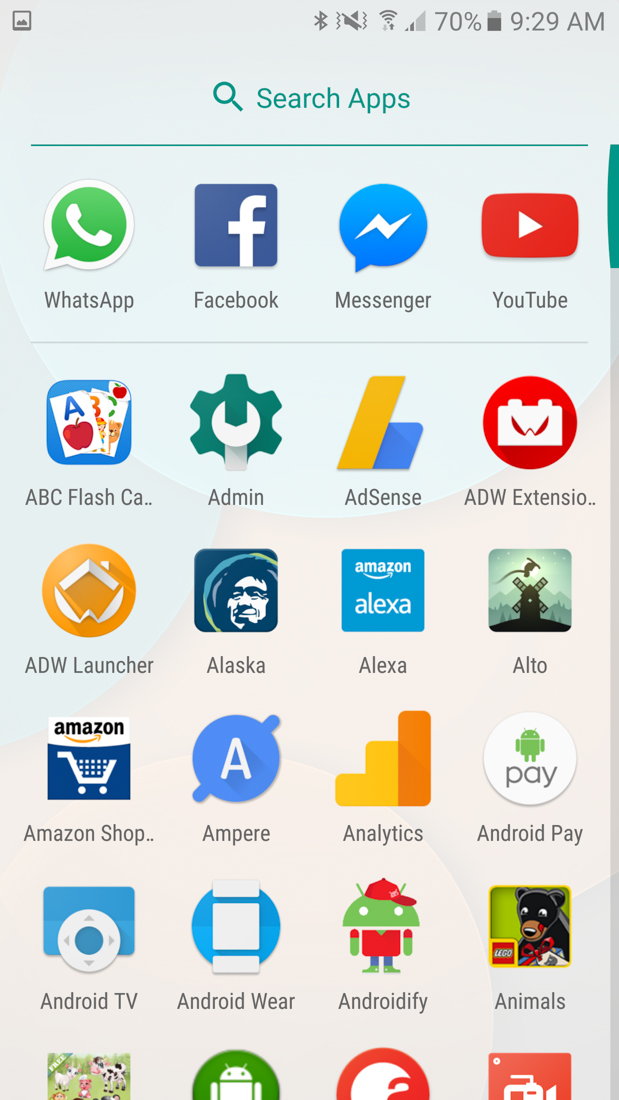A screenshot of a mobile device is depicted. At the top of the screen, standard status bar icons are displayed, including Bluetooth, a muted sound icon, a Wi-Fi signal indicator, a battery icon at 70%, and a clock showing 9:29 AM. The device's background is light gray with a turquoise-colored search bar at the top, featuring a magnifying glass icon and an underline.

Below the search bar, there are six rows of app icons, each containing four apps. In the first row are icons for WhatsApp, Facebook, Messenger, and YouTube. The second row includes ABC Flash, Admin, AdSense, and ADW Extension. The third row consists of ADW Launcher, Alaska, Alexa, and Alto. The fourth row displays Amazon Shop, Ampere, Analytics, and Android Pay. The fifth row shows apps for Android TV, Android Wear, Androidify, and Animals. In the sixth row, although the text is cut off, four icons are visible: a game featuring farm animals, an Android icon, a red and white icon with an 'A', and a red icon with a movie camera.